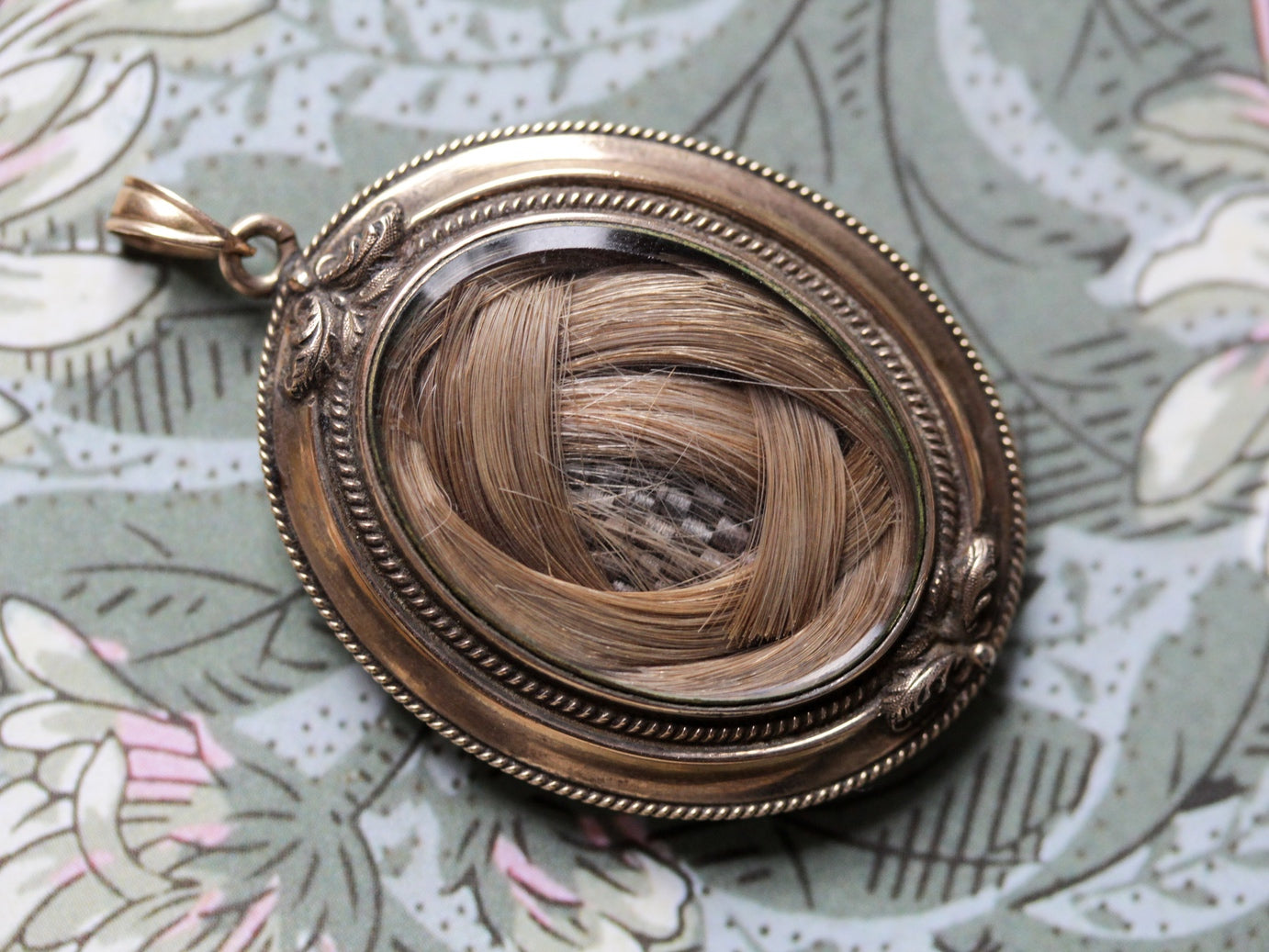The image shows a detailed photograph of a bronze or copper oval-shaped pendant, possibly a pocket keepsake or trinket. The pendant features intricate moldings at the top and bottom, resembling feathers or leaf ornamentation, and ridges along the edges similar to those on a coin. Positioned diagonally with the top towards the upper left, the pendant has a small hoop at the top, suggesting it could be used as a keychain. Inside the pendant, a lock of dark brown hair is intricately woven and rests against a surface that appears to be a green tablecloth adorned with a light blue and gray plant pattern. The image is taken from a top-down perspective in an indoor setting.